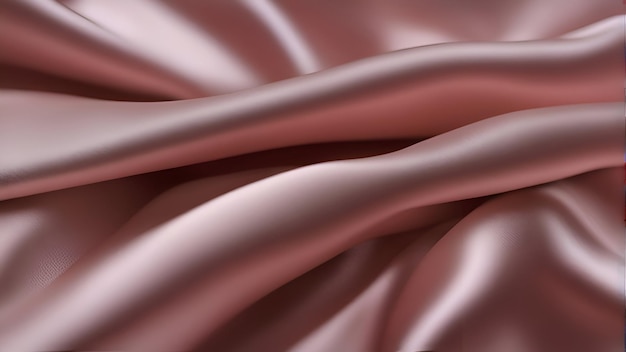The image features a full-bleed photograph of a lush, silky, pink satin fabric artfully arranged into a textured background. The background showcases a sophisticated interplay of light pinks, slightly darker pinks, mauves, and even hints of lavender or purplish-pink tones, accentuating the light and shadow within the folds. Central to the image are two prominent, almost horizontal folds framed by additional, enveloping folds at the top left and bottom right corners. These focal folds create striking contrasts of light and dark, with the shadowed areas appearing as deep maroon, enhancing the elegant, feminine feel of the fabric. The silky texture is captured vividly through the highlights on the tops of the folds, which are rendered in a nearly white, very light pink. The arrangement and folds of the satin material give the image a flowing, sophisticated, and sumptuous appearance.